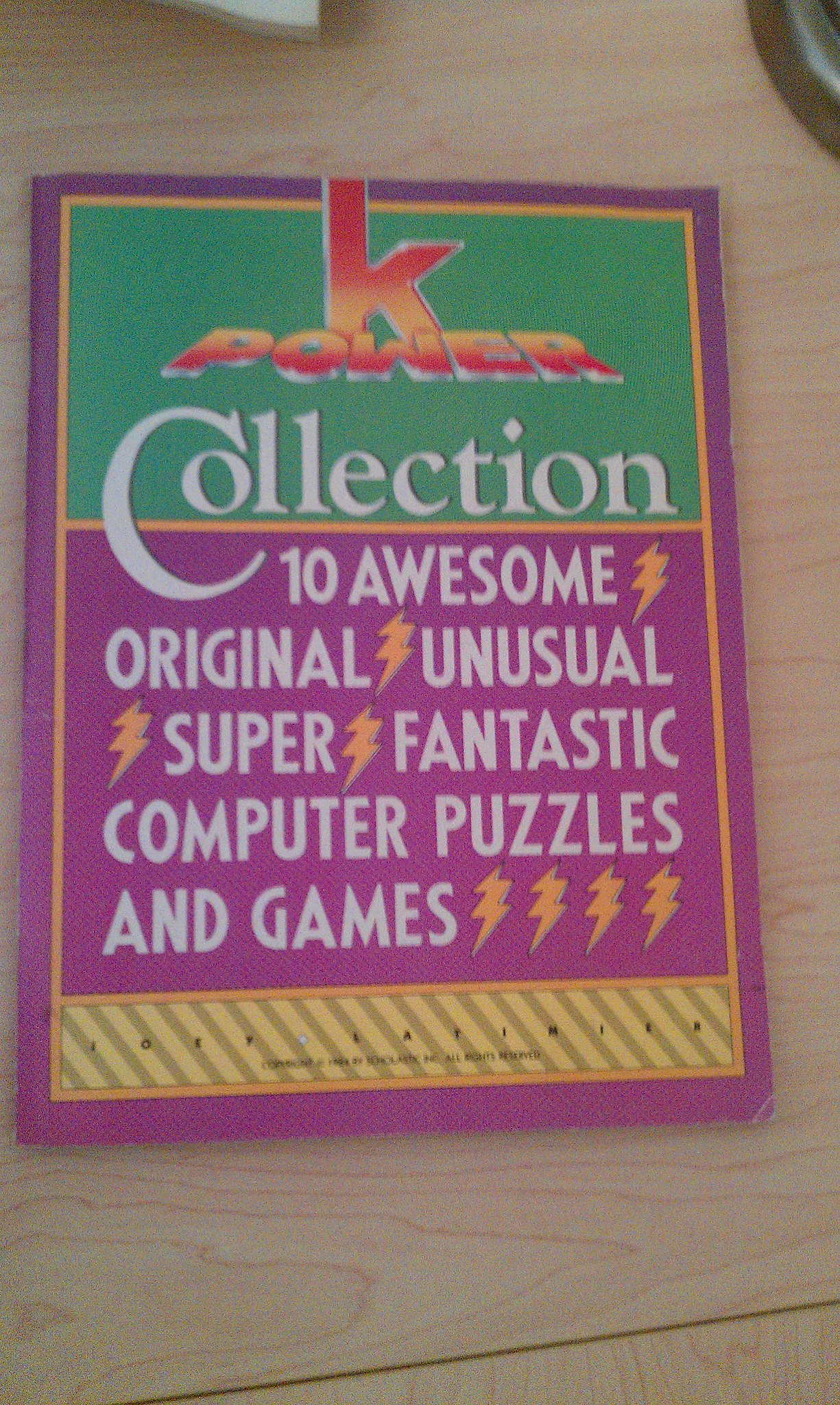This color photograph showcases a close-up of a rectangular CD case, lying atop a light-grained wooden table. The CD case features a predominantly purple background with a yellow trim around the border. At the top, there's a green block with the title "K-Power" in a 3D font that transitions from red to yellow, typical of older PowerPoint styles. Beneath this, in white letters, it reads "Collection." Below that, the text "10 Awesome, Original, Unusual, Super, Fantastic, Computer, Puzzles, and Games" is displayed, punctuated by small orange lightning bolt icons between each word grouping and four additional ones after "Games." The case is decorated with a visually striking combination of colors, including a gradient effect on the "K-Power" text and scattered orange lightning symbols. Though the lower part of the cover appears to show the author's and publisher's names, they are not legible in the image due to low resolution.